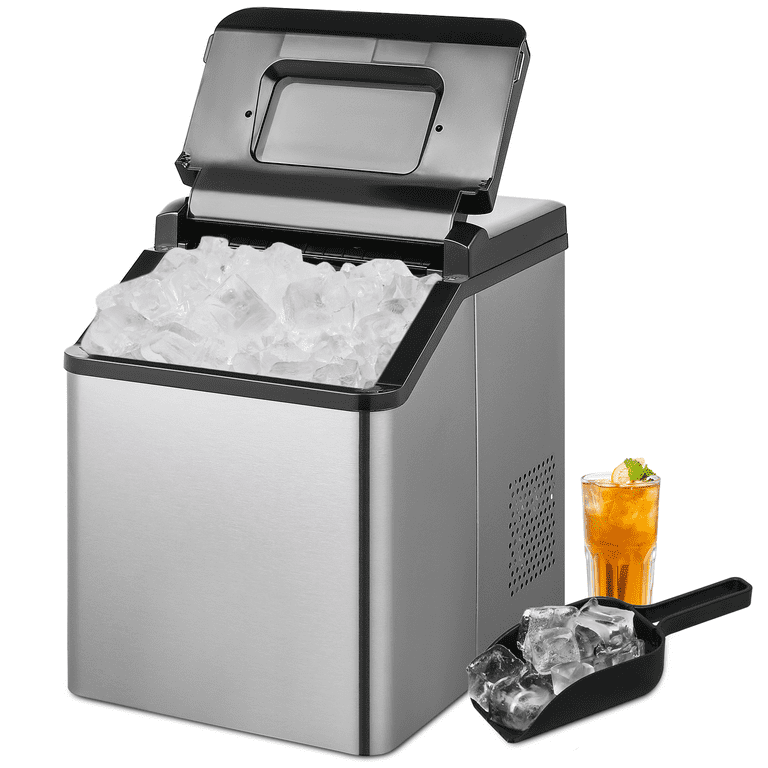The image features a portable, silver ice maker with black matte trim and a black plastic lid, which is currently open to reveal its interior brimming with ice. The machine has a distinctive flat, rectangular-shaped top lid and an air vent located on the right side. In front of the ice maker, there is a black plastic scoop filled with ice cubes, matching the color of the machine's trim. Behind the scoop, a clear glass containing a light brown, possibly iced tea beverage is visible, complete with ice cubes, a lemon slice, and a mint leaf for garnish. The photo is taken in a minimalist setting with no background or borders, focusing entirely on the ice maker and the items surrounding it.